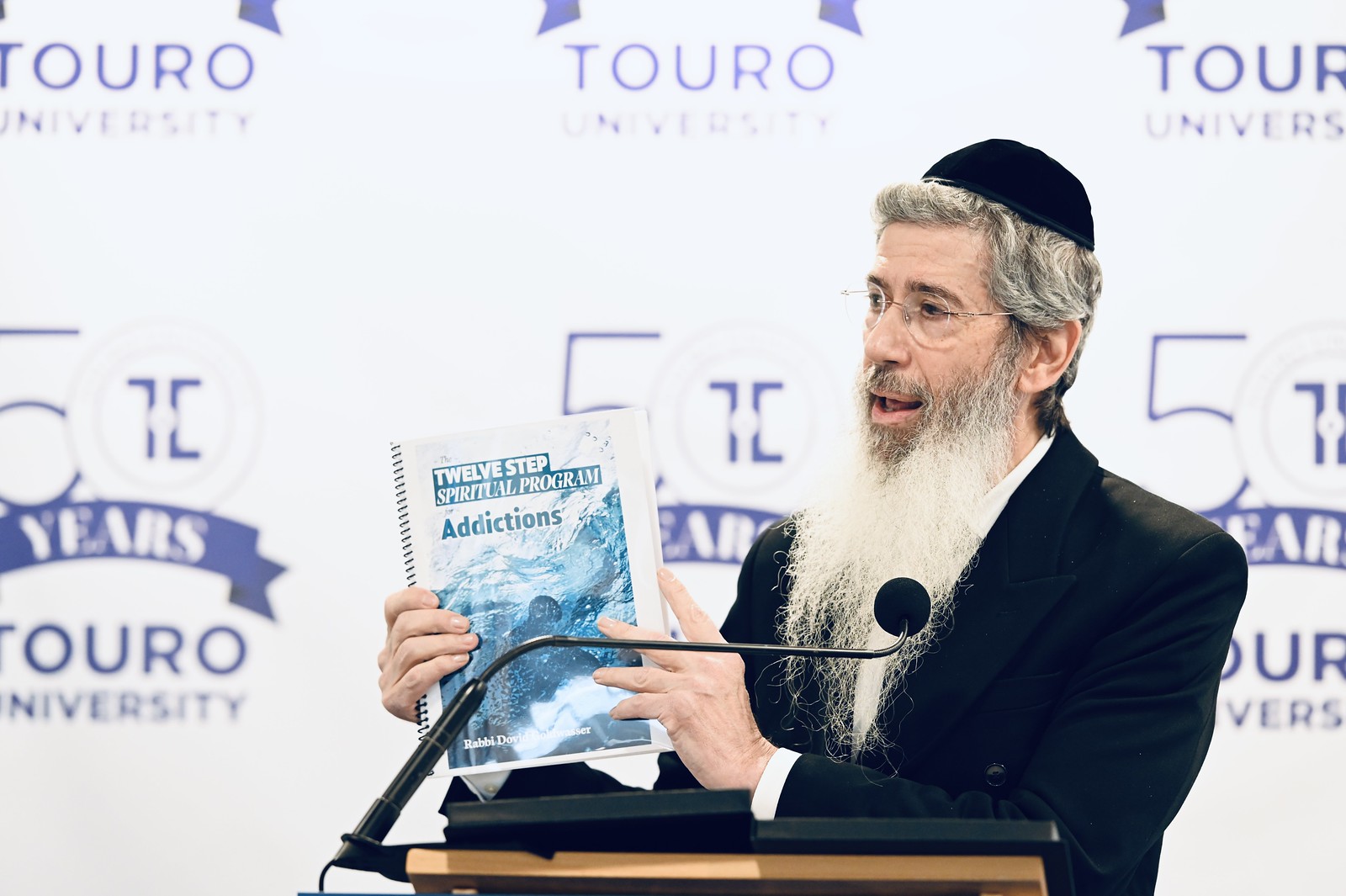In this image, an older Jewish man is seen delivering a speech or lecture on a stage, likely at a conference or seminar. He stands behind a wooden podium with black detailing, which has a microphone attached. The man, who appears to be a cleric or rabbi, has short gray hair under a black yarmulke, and a long gray-white beard reaching his chest. He wears glasses, a black blazer as part of a suit, and a white dress shirt. In his hands, he holds a prominently displayed spiral-bound book titled "12-Step Spiritual Program" with a subheading "Addictions." The book's cover is primarily white and blue, featuring an image resembling mountains and sea.

Behind him, a large banner stretches across the wall, filled with multiple logos. The background of the banner is a light blue or off-white color. The top row of the banner includes the logo "Touro University," displayed three times in purple. Lower down, a larger logo indicates "50 Years Touro University." The overall scene suggests a formal and educational setting, emphasizing the significance of the lecture.